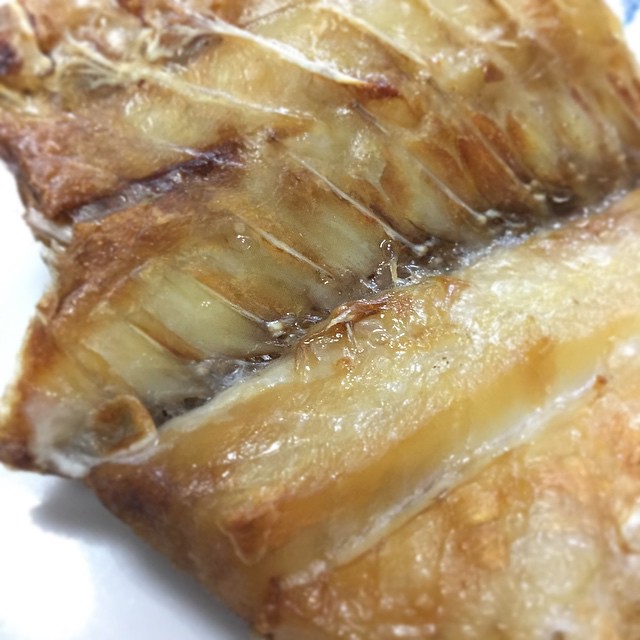The image is a highly magnified close-up of what appears to be a cooked piece of fish, displayed against a white background. The fish has a caramel-colored, gooey, and slightly sticky appearance with a glaze-like sheen. Visible are fine, brittle-looking bones and vertical segments resembling ribs, indicating it could be fish bones. There's also a darkened bone fragment towards the left center. The surface displays a mix of brown, yellow, and tan hues, with scattered translucent areas likely due to the cooking process. The lighting casts shadows below the left side of the food, adding depth to the texture and highlighting the crevices and small fissures throughout the piece.